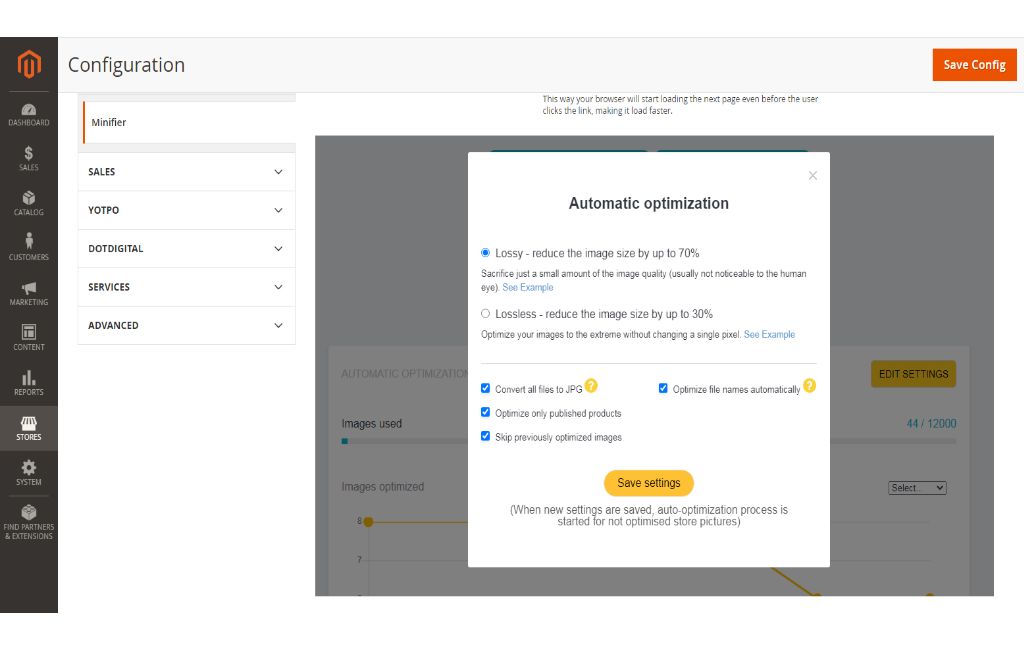The image features a configuration page from a Magento-based website, prominently displaying an automatic optimization settings pop-up. In the top left corner, the menu includes options for Dashboard, Sales, Catalog, Customers, Marketing, Content, Reports, Stores, System, and Find Partners and Extensions. The main title "Configuration" is highlighted in the sidebar.

The pop-up window offers two optimization options: "Lossy" and "Lossless." The "Lossy" option is selected, with a description indicating that it can reduce image size by up to 70% with a minor sacrifice in image quality. The "Lossless" option, also described, reduces image size by 30% without altering a single pixel.

Additional checkboxes displayed are:
- Convert all files to JPG (selected)
- Optimize filenames automatically (selected)
- Optimize only published products
- Skip previously optimized images

At the bottom of the pop-up, a yellow "Save Settings" button is visible, while an orange "Save Config" button is located at the top right corner of the main page. The footer of the pop-up includes a note stating, "When new settings are saved, the auto-optimization process is started for non-optimized store pictures."

The overall layout is clean and functional, adhering to the typical design for a settings or configuration page within a Magento admin panel.